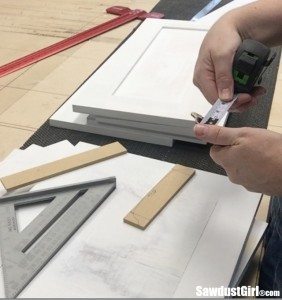This photograph captures a moment of craftsmanship in action. A pair of hands, belonging to an individual only partially visible, are meticulously engaged in measuring a piece of white wood using a measuring tape. The right hand, adorned with a wristband, holds the tape securely from the top, while the left hand steadies the measurement at the bottom. 

In the bottom right corner of the image, there is a slightly blurry yet discernible inscription reading "Sawdust Girl®" followed by the word "Calm." The background of the photograph includes a striking red metallic tool, possibly a clamp, which adds a pop of color to the predominantly neutral scene. 

To the right of the central action, a wooden table supports various tools and materials. Prominently featured in the foreground is a metal triangle-shaped tool, ready for precision tasks. Adjacent to it is a narrow piece of wood, approximately six inches long. Another shorter, thin piece of wood, around four inches long, lies to its right.

Three pieces of white wood are stacked neatly atop each other, underlining the systematic approach and tidy workspace of the craftsman. The scene radiates a sense of calm industriousness, highlighted by the careful attention to detail in measuring and arranging the materials.